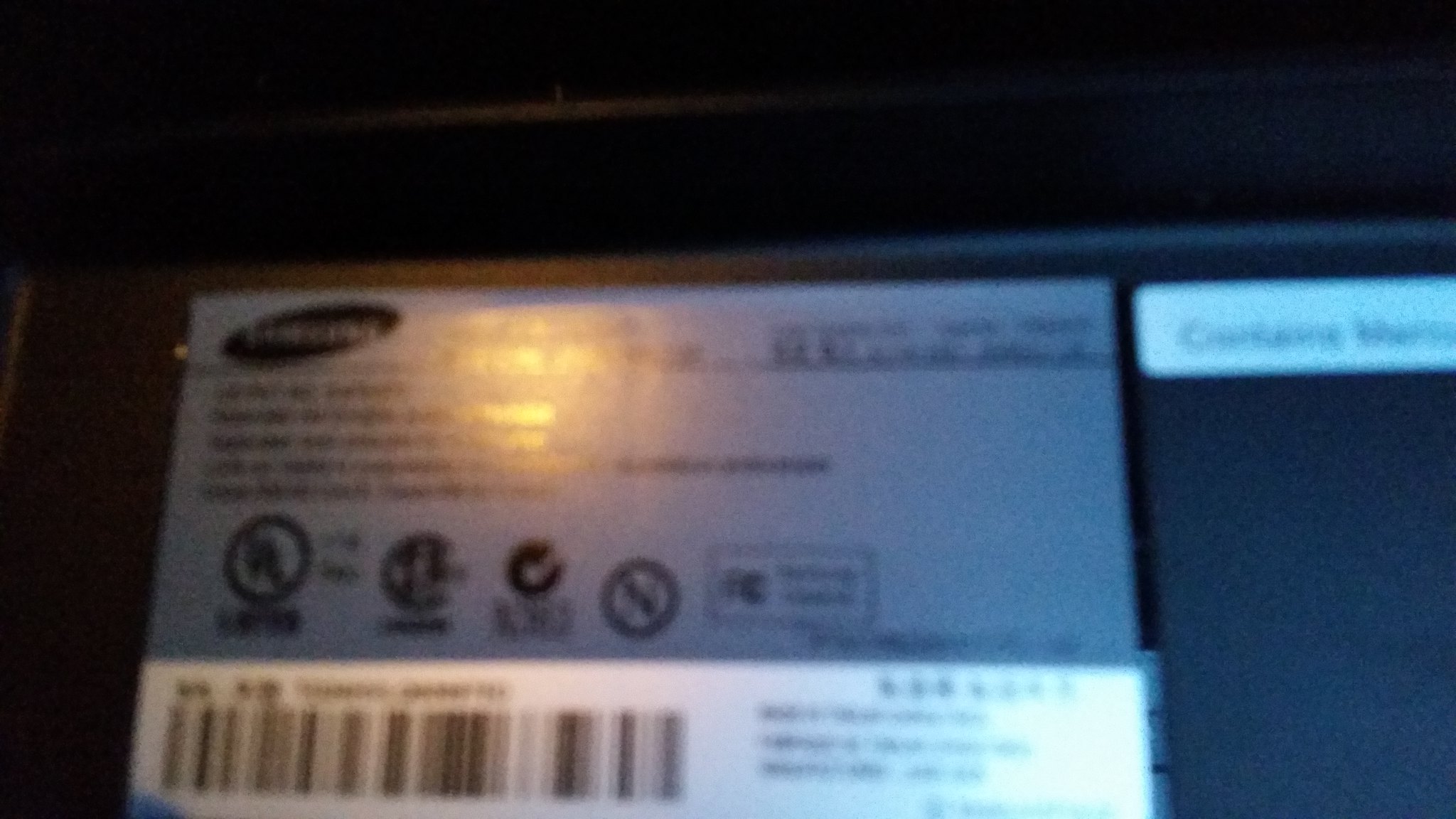This image, set against a black background, is characterized by its significant blurriness. Dominating the bottom half of the frame, approximately one inch from the left-hand corner, is a prominent white tag extending horizontally to within two inches of the right-hand side. The tag features black writing that is rendered unreadable due to the blur. Near the top left corner of this tag, there is a logo, while the bottom left corner houses a barcode. Various indistinguishable symbols are also visible on the tag. The presence of a light source further complicates the readability by causing the text to bleed together. Along the right-hand side, positioned near the top of the larger tag, a smaller white tag can be seen; it too bears black writing, which is similarly illegible due to the image’s poor clarity.